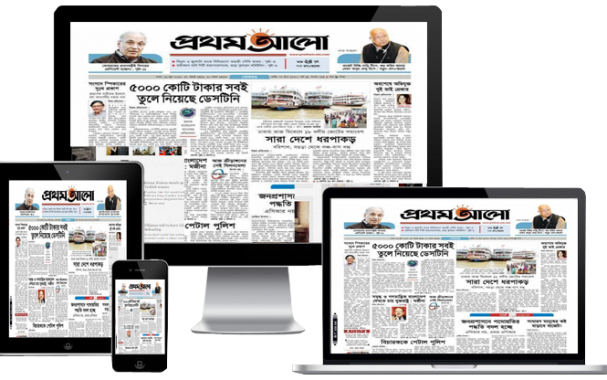The image displays a variety of electronic devices against a white background, each showcasing the same newspaper-like page in a foreign language. In the center back is a large monitor with a silver base and black bezel. This monitor displays the page prominently, which includes color images of two men at the top, surrounded by extensive text, and a photograph of ferry boats. To the left of the monitor, the same page appears on a tablet, likely an iPad. Sitting on top of this tablet, an iPhone also displays the identical page. To the right of these devices, a laptop, identified as a MacBook, is open and displaying the same page. Lastly, there is a smartphone, possibly an Android device, that also features the same newspaper page, reinforcing the recurring theme across all four devices.